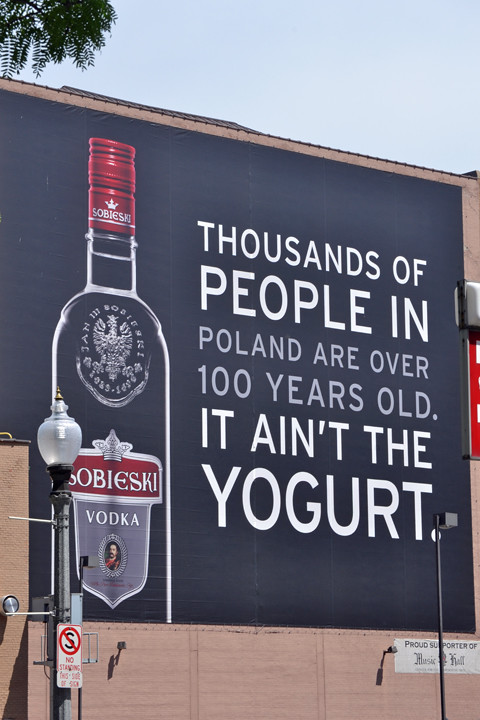This image depicts a large billboard advertisement for Sobieski vodka on the side of a tan building. The billboard showcases a bottle of Sobieski vodka with a distinctive red metal cap and a crown graphic. The background of the billboard is a very dark grey, almost black, creating a striking contrast with the bold text. The advertisement features the message in capital letters: "Thousands of people in POLAND are over 100 years old. It ain't the yogurt," with the words "Thousands of people in" and "It ain't the yogurt" in yellow, and "POLAND are over 100 years old." in white.

In the foreground, there are two prominent streetlights, and to the left of the billboard, a "No standing" sign is visible with the letter "S" crossed out. A small banner near the billboard states, "Proud supporter of Music Hall." The photo was taken during the day, as evidenced by the clear blue sky and the hint of green tree visible, adding a touch of natural color to the urban scene.